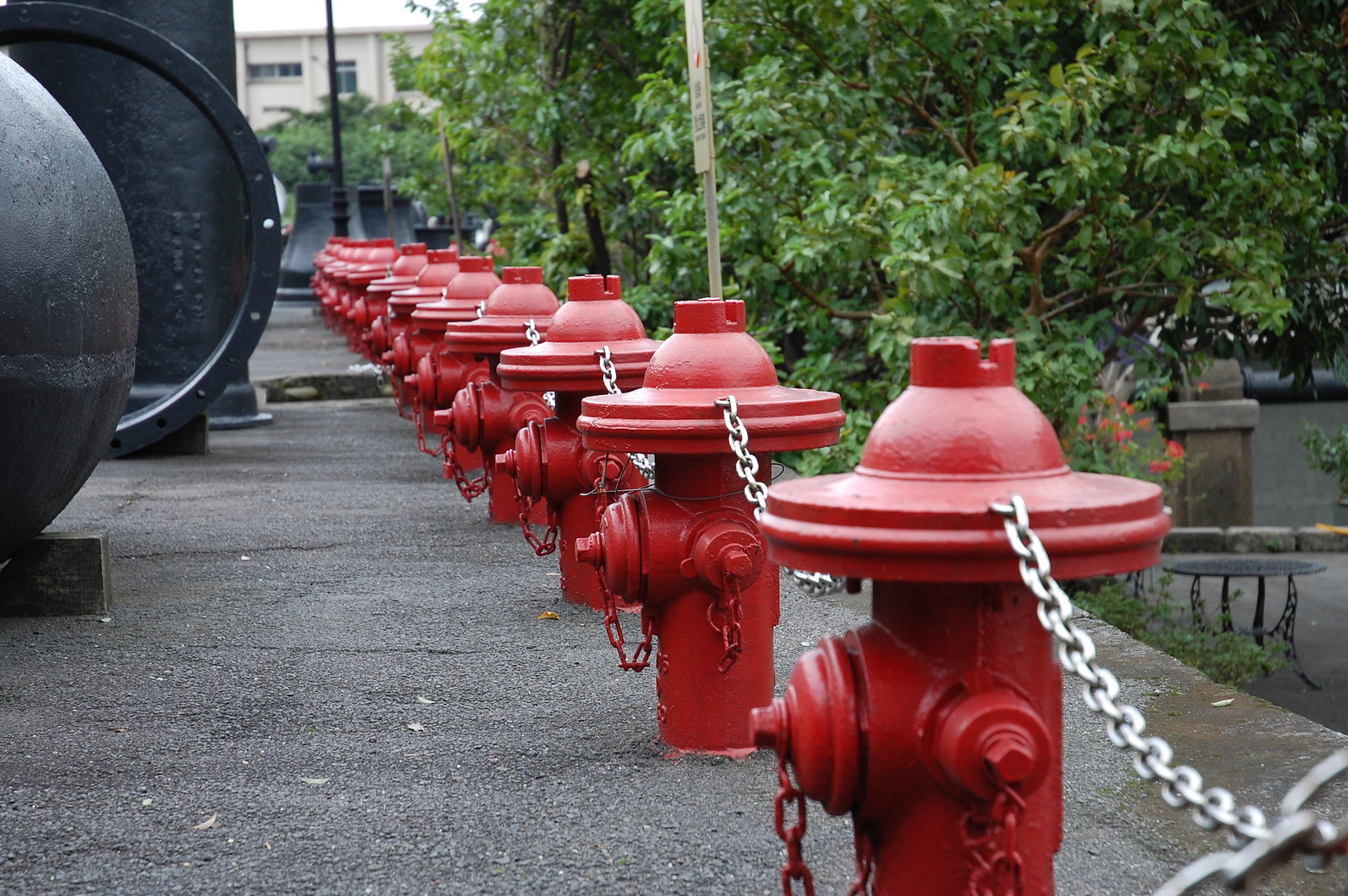The photograph depicts a scene of multiple red fire hydrants extending diagonally into the background, each connected by a silver metal chain and complemented by red chains at their bases. The hydrants are evenly spaced and positioned on a concrete floor. To the right, a line of dark green trees provides a contrasting backdrop, while to the left, there are glimpses of large, dark black sculptures. In the distance on the left, a beige building with a large black pole and a cylindrical gray piece is visible, with a tree bearing dark green leaves nearby. The area also features a black metal table and a gray wall with a tan divider topped with light gray. A pool of water is visible halfway down the image, and there is a sign behind the third fire hydrant from the foreground. The scene includes elements that become progressively smaller as they recede, giving a sense of depth and perspective.